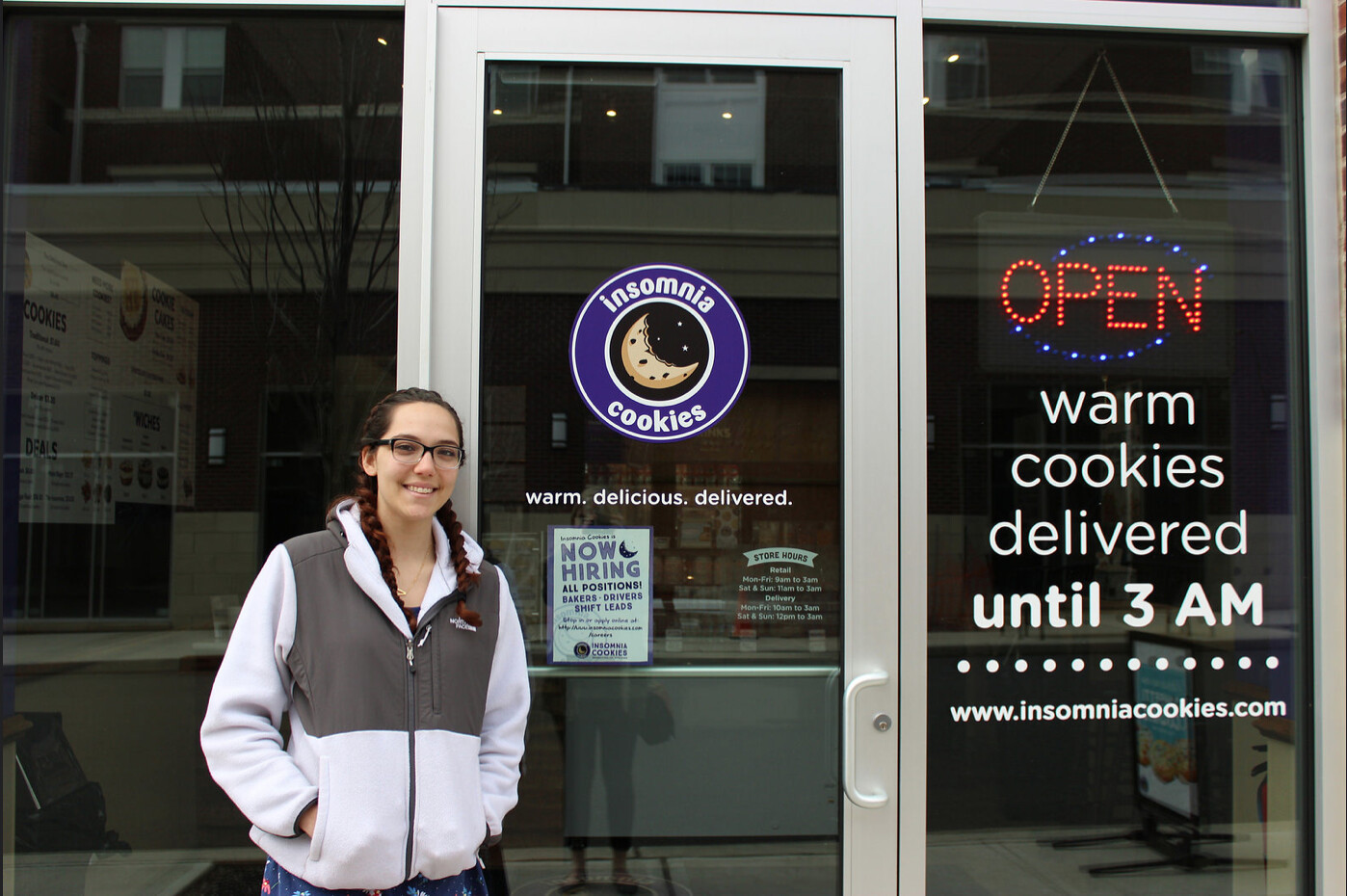A photograph captures a woman standing outside an all-glass cookie shop with prominent glass windows and doors. She's positioned to the left of the door, smiling brightly with glasses and her brown hair styled in pigtails, adorned with red highlights. She's dressed in a dark grey and white zip-up hoodie and blue jeans, with her hands casually tucked into her pockets. The door features the Insomnia Cookies logo, a blue and white emblem of a crescent moon-shaped cookie with stars, and the words, "Warm. Delicious. Delivered." A sign indicates the store is hiring for all positions. To the right of the woman, a neon LED sign glows with "OPEN" in red, surrounded by blue dots, and nearby text reads, "Warm cookies delivered until 3 a.m." along with the website address "www.insomniacookies.com". The reflection on the glass hints at the street outside, completing the vibrant and welcoming scene.